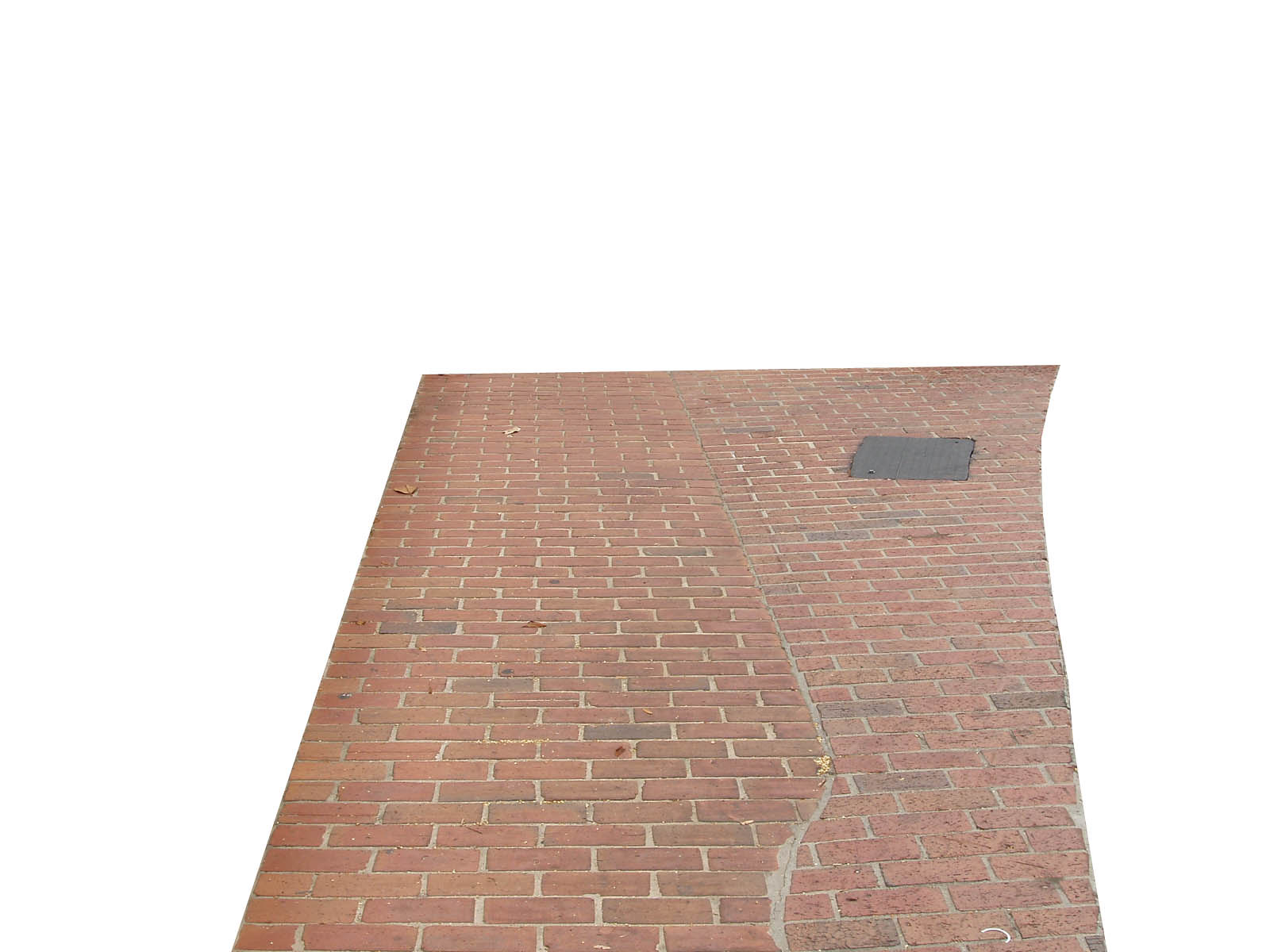The image depicts an outdoor brick pathway viewed from above, characterized by a mix of red, brownish-red, and lighter red bricks with light gray grout. The pathway has an unusual shape, curving outward on the right side and featuring sharp angles in the upper left and lower right corners. The upper left and lower right sections appear to have newer, brighter bricks with crisper lines and fresher grout. In contrast, the right side of the image shows more worn bricks and older grout. A notable black square patch is seen at the top right corner. A prominent crack runs through the center of the pathway, starting just left of center at the top, descending downward at a right angle, then curving sharply to the left in the lower part of the image. This crack has been patched with gray cement. Throughout the image, there are dried leaves scattered on the bricks, adding to the outdoor ambiance.